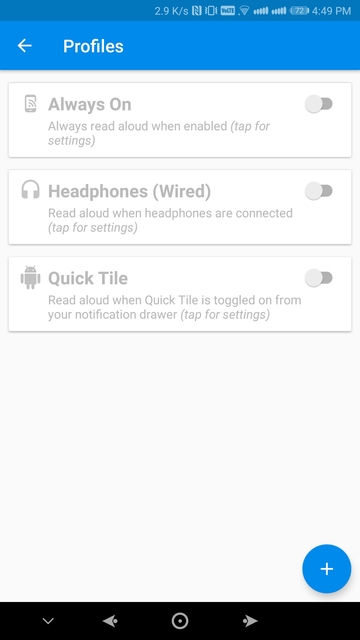This image depicts a profiles settings page on a smartphone. The top section features a blue background with the title "Profiles" and a back arrow for navigation. Below the header, the screen displays several setting options.

1. **Always On**: This setting reads "Always read aloud when enabled" and includes a "Tap for settings" option. The setting is currently turned off.
  
2. **Headphones (Wired)**: This option states "Read aloud when headphones are connected" with a similar "Tap for settings" indication. It is also turned off, as shown by the button's status.

3. **Quick Tile**: The description reads "Read aloud when quick tile is toggled on from your notification drawer" and includes a "Tap for settings" prompt. This setting is off as indicated by the gray button.

At the top of the screen, there are icons displaying battery percentage, the time, and the WIFI signal, confirming that the image is from a smartphone's settings page. 

At the bottom of the image, there is a circular blue button with a plus sign, likely for adding additional settings or adjustments. The bottom bar contains four buttons: a down arrow, a back button, a center home circle, and a forward-facing arrow.